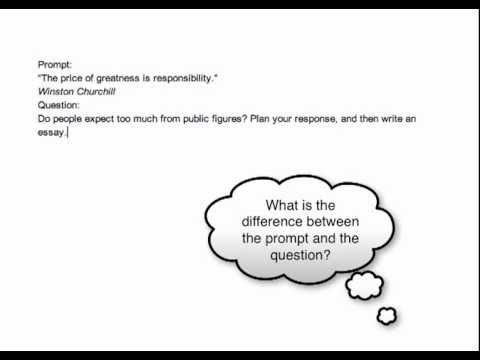The image is a horizontally oriented rectangular slide designed for teaching grammar. It features a thick black border along the top and bottom with a thin black line on the right side, leaving the left side without any border. The slide's quality is notably low, with pixelated and somewhat blurry text. In the upper left corner, the text begins with "Prompt," followed by a quote: "The price of greatness is responsibility. — Winston Churchill." Below that, closer to the lower right corner, is another block of text labeled "Question: Do people expect too much from public figures? Plan your response and then write an essay." In the bottom right corner, within a cloud-shaped speech bubble stylized to resemble a conversation balloon from a cartoon, the text reads, “What is the difference between the prompt and the question?” The overall color scheme of the image is limited to black, white, and gray, with substantial blank space surrounding the text elements. The slide appears to be illustrating or prompting a discussion on the distinct roles of prompts and questions in assignments.